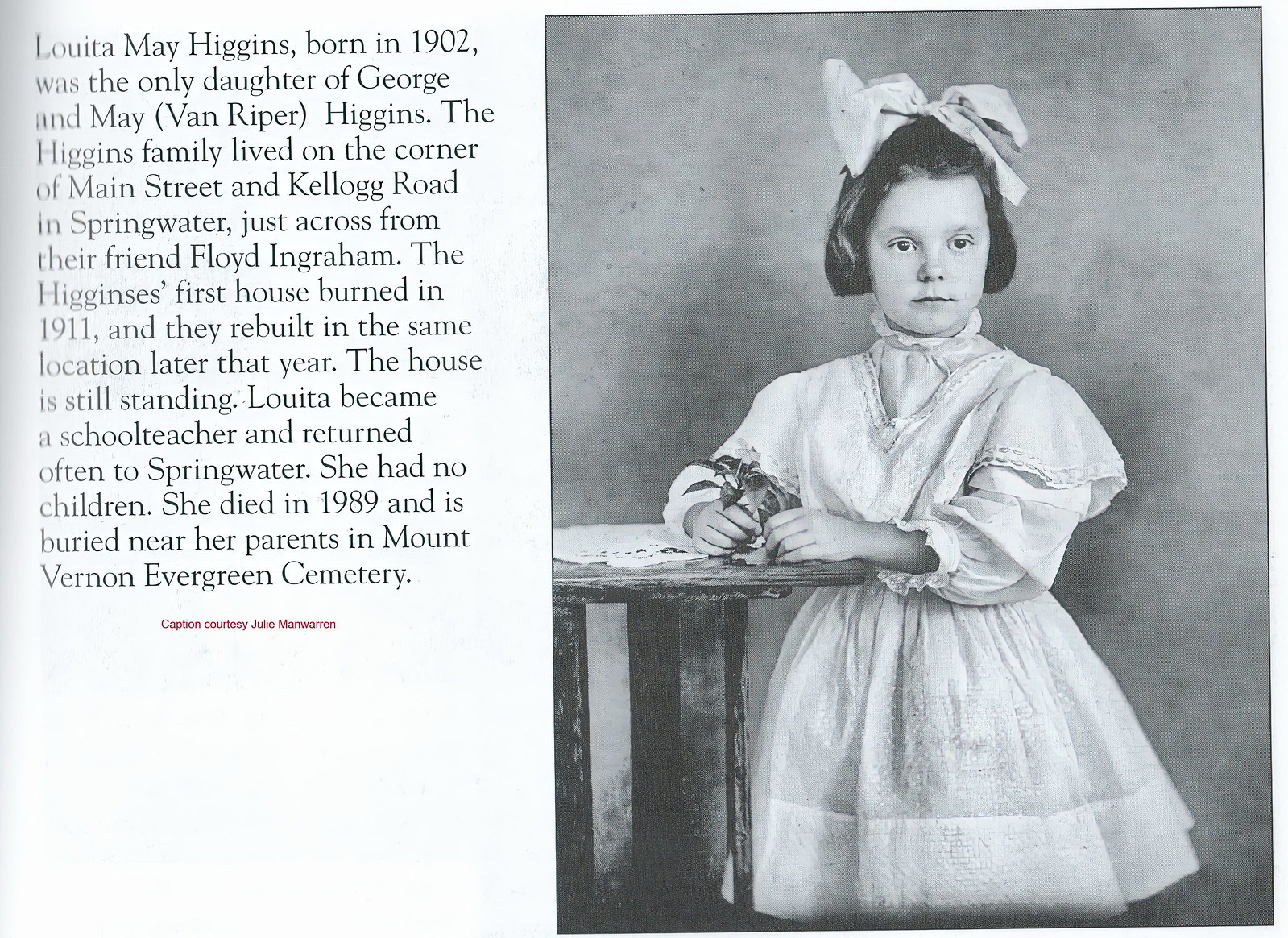The image depicts an obituary card in black and white with a rectangular layout, divided into two panels. The left panel, occupying about 40% of the image, features a white background with black text detailing the life of Luida Mae Higgins. Born in 1902, she was the only daughter of George and Mary Van Ripper Higgins. The family resided at the corner of Main Street and Kellogg Road in Springwater, across from their friend Floyd Ingraham (or Ingram). Their first house, which burned down in 1911, was rebuilt later that year and still stands. Luida pursued a career as a schoolteacher and returned to Springwater often. She had no children, passed away in 1989, and was buried near her parents in Mount Vernon Evergreen Cemetery. Below this information, in small red lettering, is the note: "Caption Courtesy of Julie [something]."

The right panel, which takes up 60% of the image, features a black and white sketch of a young girl with dark hair adorned with a white bow. She is wearing a white dress and is standing with her hands on a table, looking directly at the viewer. The background is composed of varying shades of gray.